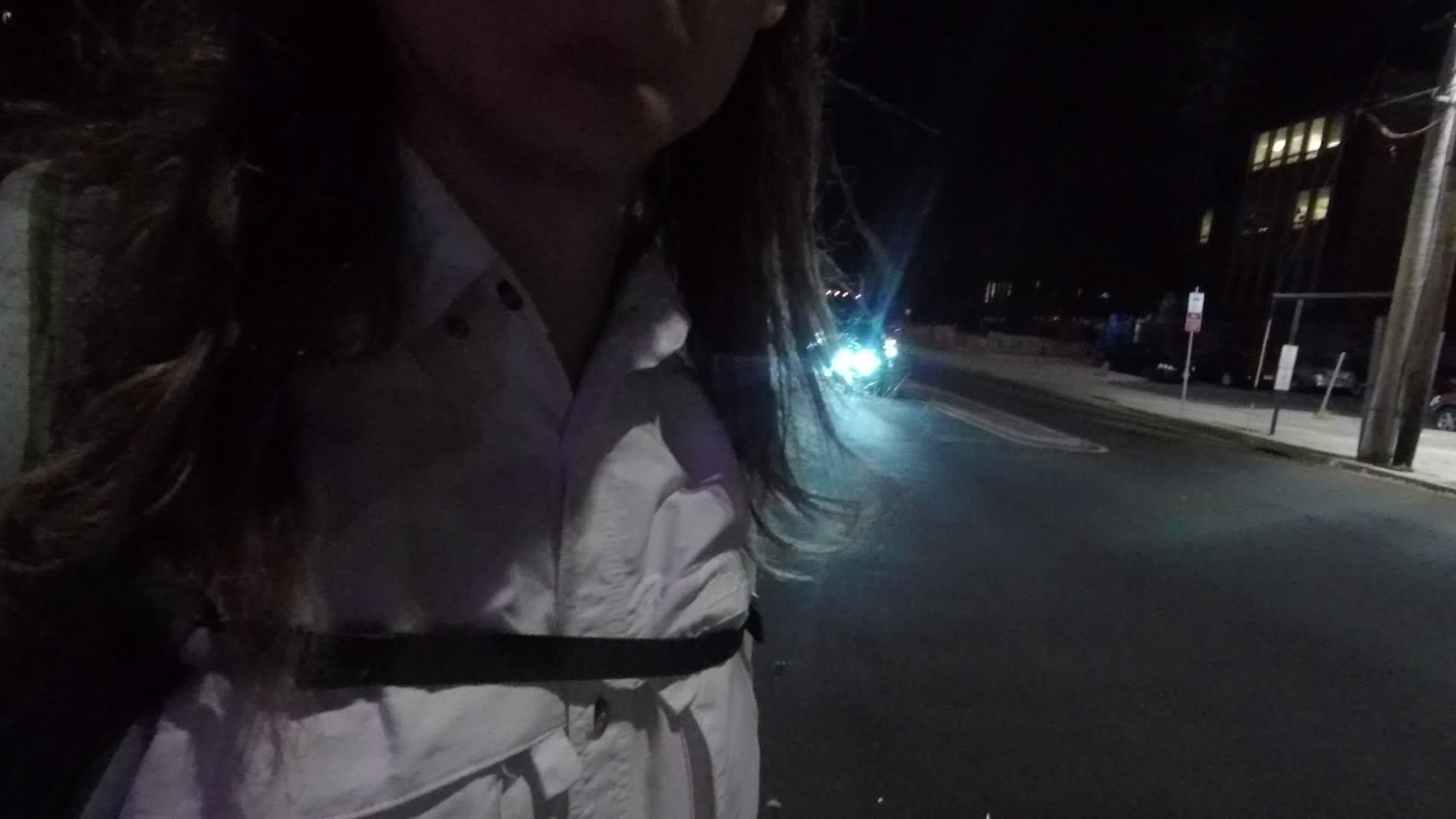This color photograph, taken at night, reveals a close-up, partial view of a woman standing on a sidewalk by a road. The frame captures her chin down to her chest, with her head and lower torso cropped out. She has long, flowing brown hair that appears to be illuminated from behind by a car's headlight, highlighting the strands and texture. She is dressed in a white, wrinkled collared shirt with the top button unbuttoned, revealing pockets on both sides of her chest. She wears a backpack, with the strap visible on the left side behind her hair and a thin black chest strap across her torso. Her positioning fills the left side of the horizontally oriented image, while the right side includes a road, a concrete curb, a large metal pole, two street signs, and a building with illuminated windows on the top floor. The scene is set in darkness, marked by the presence of car headlights and streetlights that add depth to the backdrop.